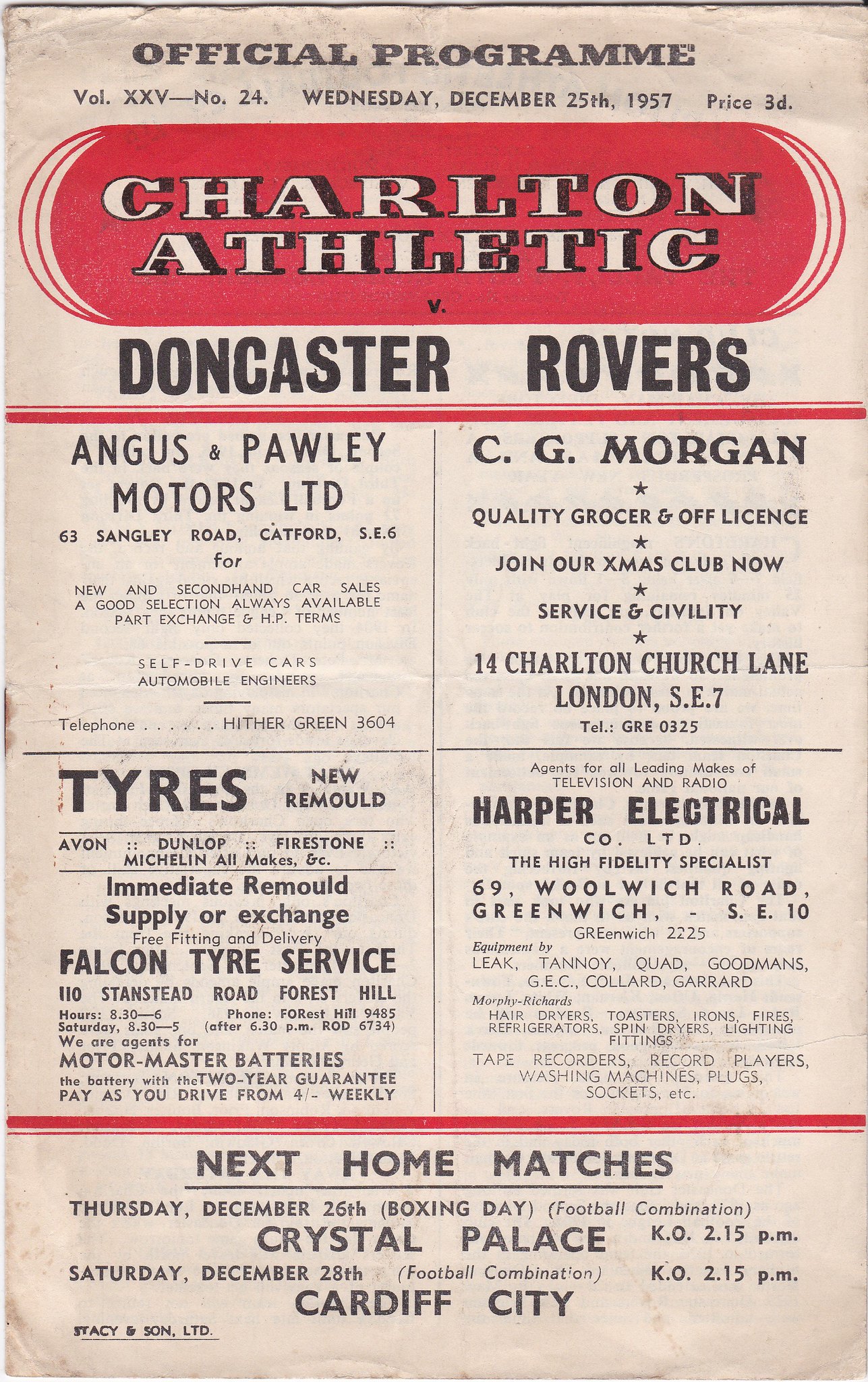This image is an aged and slightly wrinkled official program from 1957 for a soccer match between Charlton Athletic and Doncaster Rovers, printed on a light pink to off-white background. At the top, in red letters, it reads "Official Program," with "Charlton Athletic" immediately below. The central section is divided into quadrants featuring various advertisements. 

In the top left quadrant, there's an ad for Angus and Pauly Motors Ltd, and to the right, an ad for C.G. Morgan, Quality Grocer and Off License. The second row features an ad for New Remold Tires on the left and Harper Electrical Co., the high fidelity specialist, on the right. Below these ads, a red line separates them from the bottom section, which provides information about upcoming home matches, including encounters against Crystal Palace on Thursday, December 26th (Boxing Day), and against Cardiff City on Saturday, December 28th (Football Combination).

The program denotes its volume and issue number as Volume 25, Number 24, and specifically dates it to Wednesday, December 1957. Notably, at the bottom, there are additional advertisements like "Yacy and Son Ltd." The entire document evokes a sense of nostalgia, reflecting its era through its content and appearance.